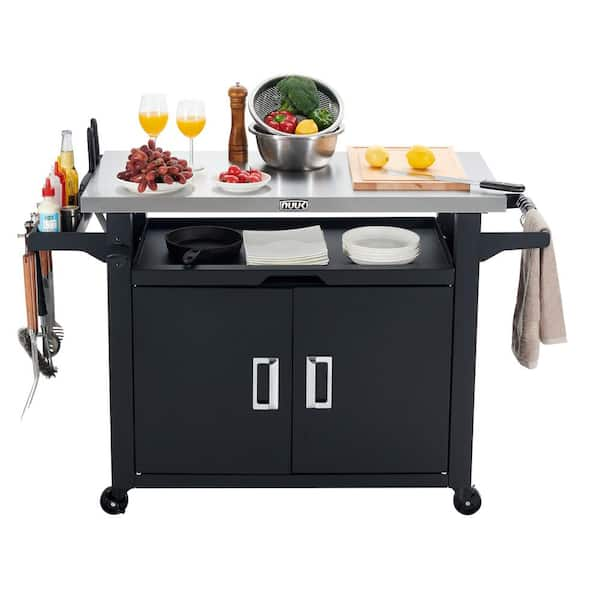This color photograph features a gray metal rolling outdoor kitchen island with a versatile design. The base of the cart consists of black-painted cabinets with silver handles, including a lower shelf that holds an iron cast skillet, paper plates, and napkins. The cart has a silver countertop adorned with an array of items: a bowl of vegetables, a wooden pepper grinder, two lemons on a wooden cutting board with a knife, and two wine glasses filled with an orange-colored beverage. To the right side of the cart, a towel is draped over a handle, while the left side has hanging pegs for various grilling utensils and barbecue tools. Additionally, there's a small section for condiments, holding bottles and jars. The countertop also features plates with diverse foods, bowls, and another smaller bowl of fruit indicating a well-prepared setup for outdoor dining or cooking.